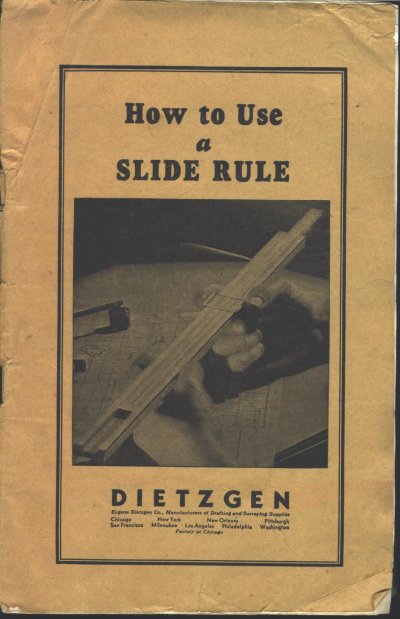The photograph showcases the cover of an old, worn-out paperback book titled "How to Use a Slide Rule" by Dietzgen. The cover, primarily beige in color, features a prominent black vertical rectangle centered within it. At the top of this rectangle, the title is clearly displayed in bold black text. Just below the title, there is a black-and-white photograph of a right hand holding a slide rule at an angle, suggesting a practical application. Underneath the photograph, the author’s name "DIETZGEN" is printed in capital letters, followed by smaller black text listing several city names, such as Chicago, New York, New Orleans, Pittsburgh, San Francisco, Milwaukee, Los Angeles, Philadelphia, and Washington, among others. The image has an aged appearance, with the book occupying the entirety of the photo, set against a dark background that accentuates its antiquated look.